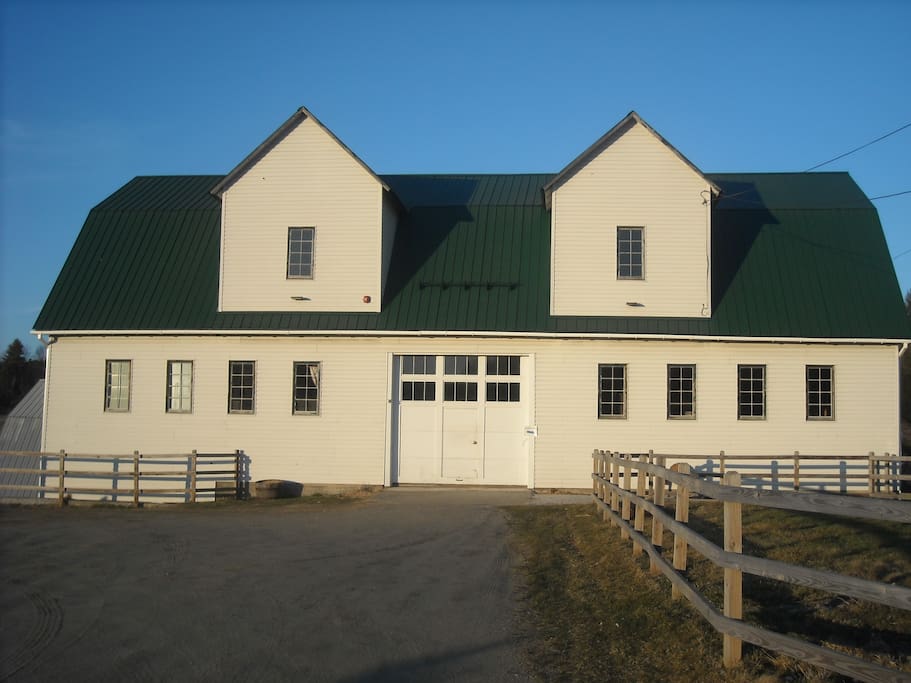The image depicts a modern, off-white or cream-colored barn with a distinctive green metal roof that slopes upward and then curves back down. The barn features two eaves on the roof, each shaped like a small house with a vertical rectangular window, meeting at triangular points. The main part of the barn has a wide, imposing central door designed like a garage door, which includes three rows of windows at the top, allowing light to enter. Flanking the central door are four vertical rectangular windows that span horizontally across both sides of the structure.

Surrounding the barn is a brown wooden plank fence, composed of three horizontal planks connected by vertical poles. This fence is positioned to the right of the barn, while the left side appears open, and it extends along the driveway leading up to the barn. The ground in front of the barn consists of gray dirt that forms a pathway. The bright blue sky in the background is strikingly clear, devoid of any clouds, emphasizing the daylight setting and highlighting the barn's detailed structure, from its large, double-door entrance to the multiple windows and architectural elements.